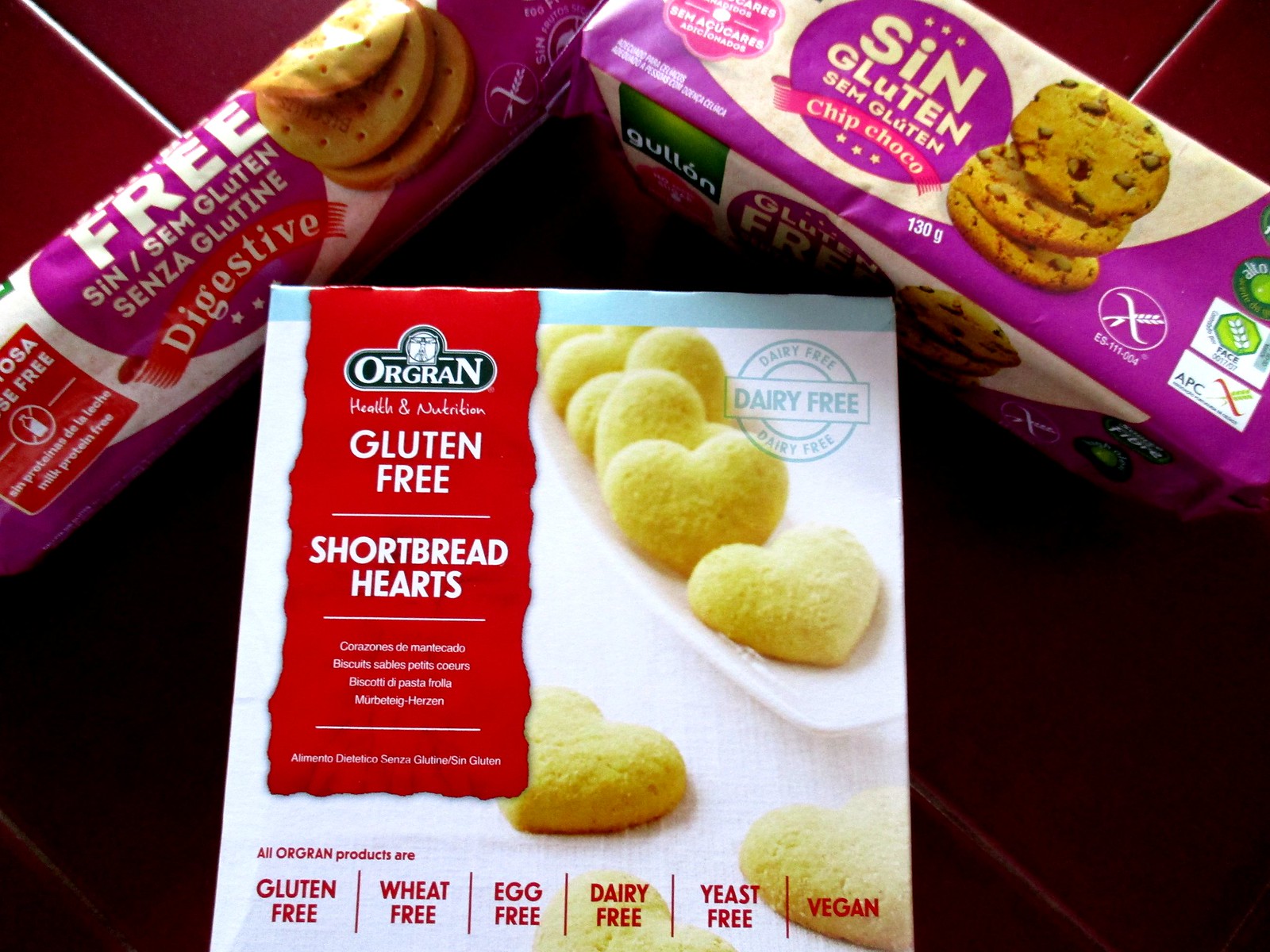The image depicts three different packs of cookies arranged on a surface made up of ceramic-like red tiles with white grouting in between. The top left package, encased in thin plastic material, features purple and white colors and displays the text "Free Syn Sem Gluten Senza Gluten Digestive," accompanied by images of cookies. A small warning label indicates that the product is free from milk proteins. 

In the center lies a box made of cardboard, with a distinctive red tag that reads "Gluten-Free Shortbread Hearts." This package prominently displays heart-shaped cookies that are a whitish vanilla color and includes multiple allergy-friendly labels stating "gluten-free, wheat-free, egg-free, dairy-free, yeast-free, vegan."

On the right, there is a rectangular-shaped plastic container showcasing chocolate chip cookies. This package also carries a purple and white theme, with a label that reads "Syn Gluten Sem Gluten Chip Choco." The cookies inside are visible through the packaging, stacked neatly in rows. 

Overall, the picture captures a variety of gluten-free baked goods, each in distinct packaging, set against a tiled indoor surface.